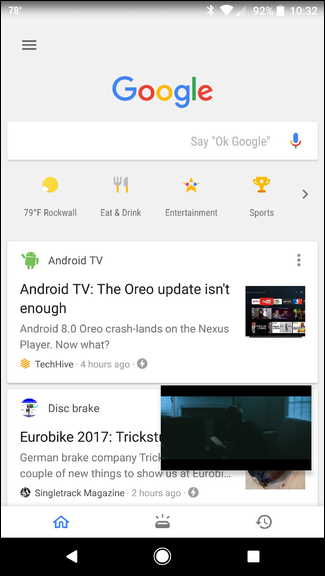The image is a screenshot captured from a mobile device, displaying a Google search window. The background is predominantly white, imparting a clean and minimalistic appearance. At the very top of the image, the colorful Google logo is prominently featured, showcasing its familiar blue, red, yellow, green, blue, and red letters.

Directly beneath the logo is the Google search bar, with the phrase "Say 'Ok Google'" written within it. The search bar also includes a microphone icon, colored in blue and red, set against the bar's white background.

Below the search bar, there are several categorized search options, each accompanied by a corresponding icon. The categories listed are "79 degree rockfall," "Eat and Drink," "Entertainment," and "Sports."

Further down, there is a white rectangular frame or window. Inside this window, the text "Android TV" is displayed, accompanied by a small green Android icon to the left of the words. Below this, the text continues in black, stating, "The Oreo update isn't enough."